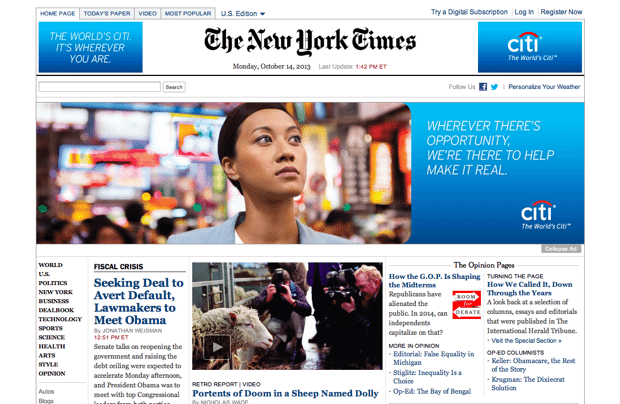**Screenshot from The New York Times Homepage - October 14, 2013**

This detailed screenshot captures the homepage of The New York Times, dated Monday, October 14, 2013, and last updated at 1:42 PM Eastern Time. At the top of the page, navigation tabs are visible, including options for "Homepage," "Today's Paper," "Video," "Most Popular," and "U.S. Edition," with "Homepage" currently selected.

Adjacent to these tabs on the right side, a prominent blue rectangle showcases the slogan "City: The World City." Directly beneath this banner, a search bar is provided, followed by social media prompts to "Follow us on Facebook or Twitter" and an option to "Personalize Your Weather."

Dominating the center of the screen, a vibrant image features a person with dark skin, almond-shaped eyes, and closely cropped dark hair, dressed in a gray suit and white shirt. The individual stands against a brightly lit backdrop, suggesting a lively environment such as a restaurant or mall. Overlaying this image is the text: "Wherever there is opportunity, we're there to help make it real. City: The World City."

The left column of the page lists various sections of the paper, including "World," "U.S.," "Politics," "New York," "Business," "DealBook," "Technology," "Sports," "Science," "Health," "Arts," "Style," "Opinion," "Autos," and "Blogs."

Highlighted articles include a headline on the fiscal crisis titled "Seeking Deal to Avert Default, Lawmakers to Meet Obama," accompanied by a striking photograph of a sheep surrounded by photographers. Beneath this article, a "Retro Report Video" caption reads, "Portents of Doom, and a Sheep Named Dolly."

On the right side, "The Opinion Pages" section features discussions on "How the GOP is Shaping the Midterms" and "Turning the Page: How We Called It Down Through the Years," providing readers with analytical content.

This sophisticated layout and diverse content reflect The New York Times' commitment to delivering comprehensive news and insightful opinions to its global readership.